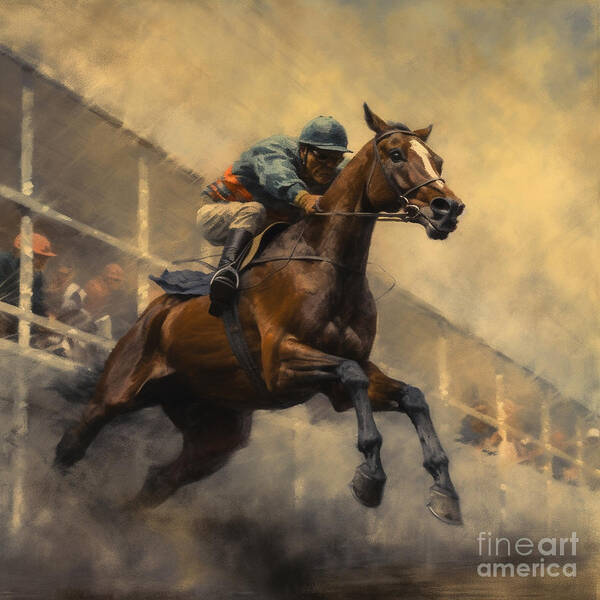A dynamic and detailed artwork captures a thrilling moment of a jockey riding a leaping brown horse, centrally positioned in the image. The jockey, sporting a blue helmet, a long-sleeve blue shirt with an orange stripe, gray pants, and black boots, is hunched over, aiding the horse's jump. The horse, with all legs off the ground, appears to be bursting through a smoky, murky background that features a vast stadium arena filled with spectators. Its distinguishing white patch runs down the center of its face, contrasting with its black bridle and partially black legs. The sky overhead is cloudy with shades of whitish-blue, adding to the dramatic ambiance. In the bottom right corner, gray text reads "Fine Art America," lending an additional layer of intrigue to this captivating scene.